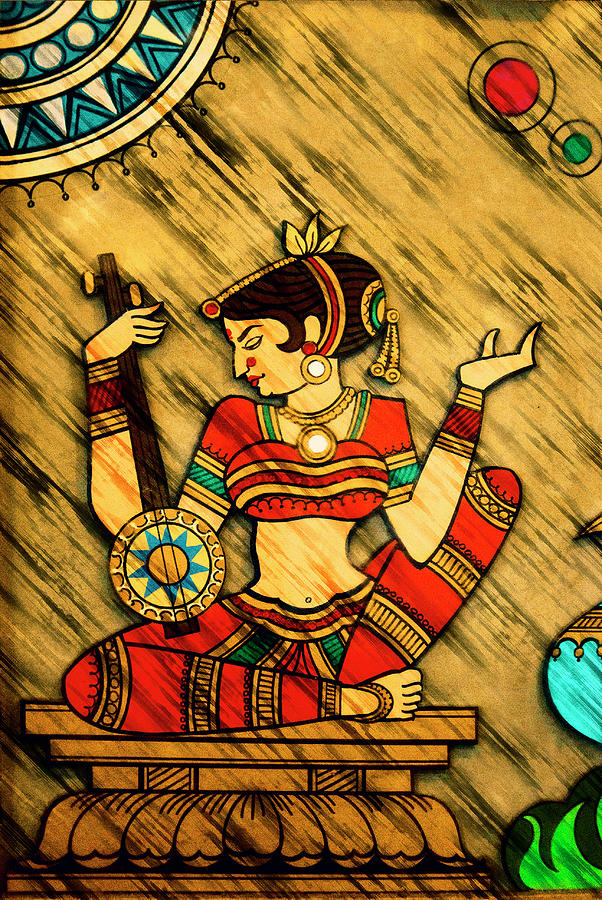The image showcases a detailed Indian artwork on a wooden background, characterized by darker, streak-like patterns that appear burnt or painted. In the top left corner, there's a golden sun with blue layers, while the top right corner features a red circle outlined in black, with a smaller green center encased within a black ring. Along the right edge, a blue crystal bowl with green flames beneath it can be seen.

Prominently displayed on an intricately carved wooden stool is a woman adorned in traditional, vibrant attire. She wears a midriff-baring British orange top, combined with red, green, and gold pants that include turquoise green and golden lines. Her outfit is complemented by extensive jewelry, including a ribbon in her dark, pulled-back hair and a red bindi on her forehead. She has red earrings, red lipstick, and gold ornaments decorating her head and body.

The woman is in the act of playing a string instrument resembling a banjo, with a dark wooden neck and circular body. One arm is raised, adding a dynamic element to the scene. The background above her is adorned with star shapes in turquoise blue with gold centers, and additional red and green circular patterns around her. The artwork's overall tone is enhanced by a yellowish hue, giving the piece a rich, warm feel.